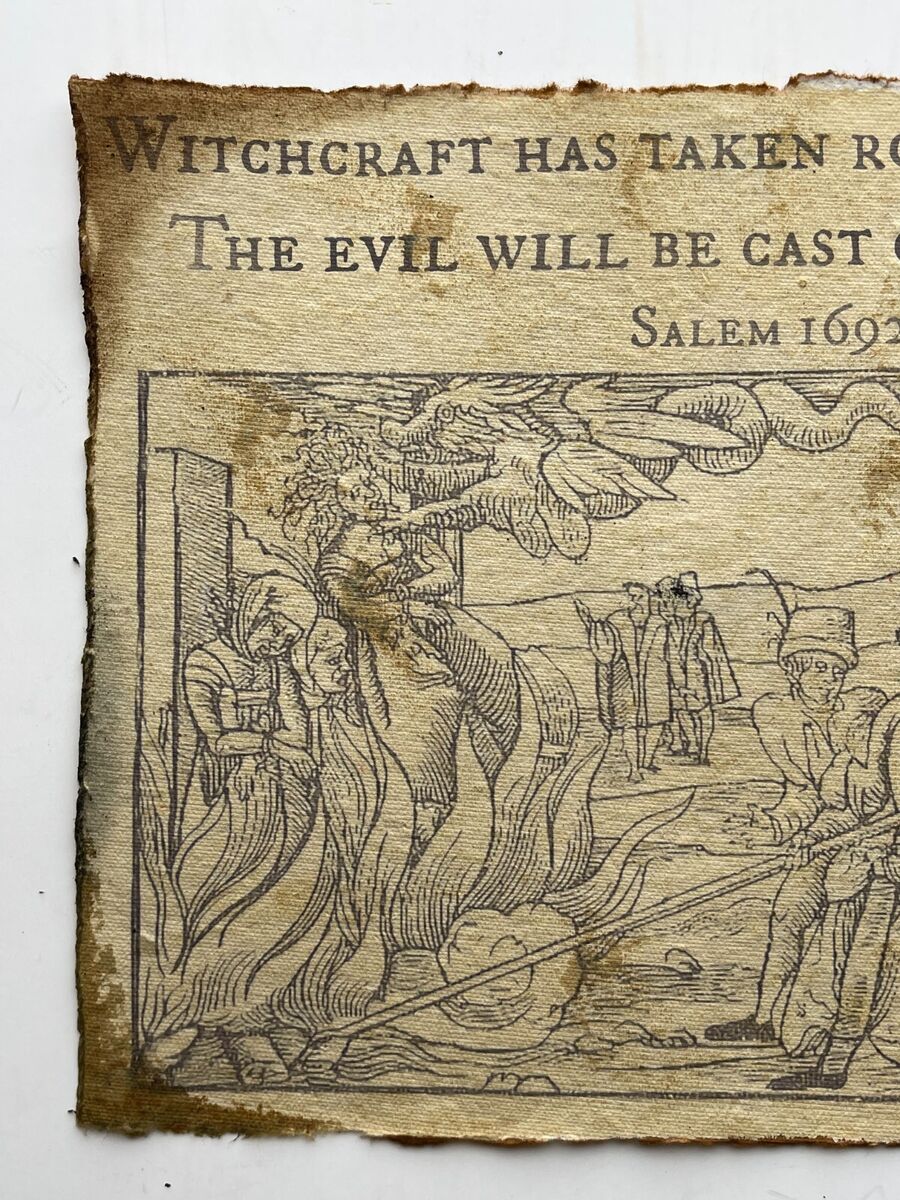This image appears to be a photograph of an old, partially visible page from a tattered book or an aged piece of parchment. The page is significantly faded, with edges that appear water-damaged or burnt, giving it an authentic antique look. The text that is visible reads: "Witchcraft has taken... The evil will be cast... Salem 1692," likely completing the phrases "Witchcraft has taken root" and "The evil will be cast out." The text is printed in black on a tan-colored paper.

The illustration on the page, reminiscent of a historical woodcut etching, depicts a grim scene from the Salem witch trials. In the center, several women are bound to stakes with flames rising around them. To the right, a man wearing a hat is using a long tool to stoke the fire. Overhead, a dragon soars through the sky, adding a fantastical element to the image, while several onlookers stand in the background, observing the horrifying scene with a casual demeanor. The illustration captures the harsh and brutal imagery associated with the witch trials of 1692.